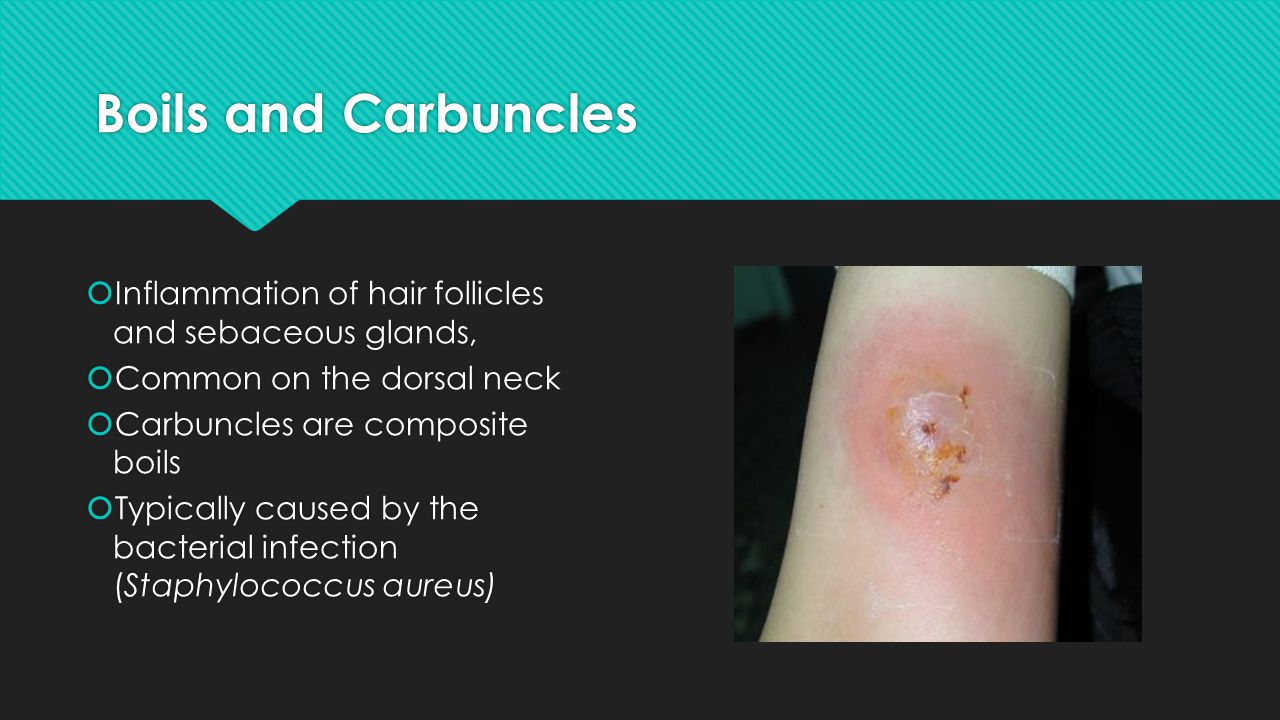This horizontal rectangular PowerPoint slide features a detailed medical presentation on boils and carbuncles. The slide has a predominantly black background with a turquoise stripe at the top, which includes a small triangle jutting out on the left side. In white font atop this stripe, the title "Boils and Carbuncles" is prominently displayed. 

Beneath this stripe, on the right side of the slide, is a close-up photograph of a person's arm showing a skincare issue characterized by light pink scabbing, red spots, orange spots, and a white blister in the center. A small depiction of a bandage is visible in the upper right-hand corner of the affected area.

To the left of this image, a set of informational bullet points, denoted by green circles, is listed in white font. These points explain that boils and carbuncles involve inflammation of hair follicles and sebaceous glands, are common on the dorsal neck, and identify carbuncles as composite boils typically caused by the bacterial infection Staphylococcus aureus. The text features the scientific name of the bacteria in italics.

An arrow, also in turquoise, points from the title section down towards the bullet points, guiding the viewer's attention to the important textual information presented alongside the medical depiction.